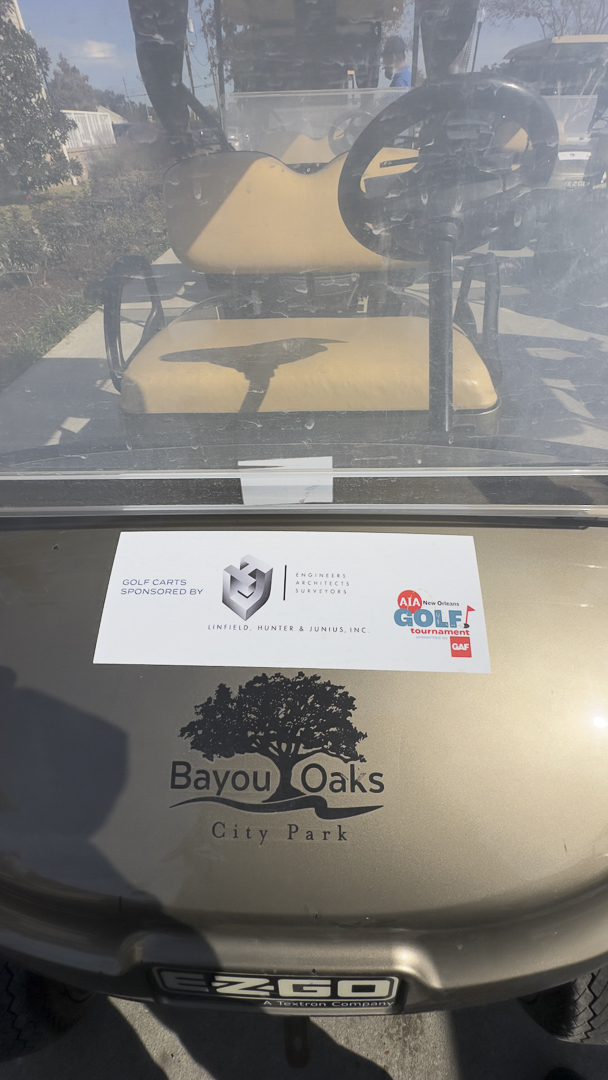The image captures a close-up front view of a golf cart at Bayou Oaks City Park, emphasizing the details seen through and on the windshield. The body of the golf cart is a metallic silver or gray color, with a prominent emblem on the front hood featuring a large black tree and the text "Bayou Oaks City Park." This golf cart appears to be participating in a golf tournament, as indicated by additional emblems and signs. One of these signs, somewhat hard to read due to small gray lettering on a white background, indicates sponsorship by Linfield, Hunter and Junius Incorporated. Another emblem in blue and red reads "GAF Golf Tournament." The windshield is slightly dirty, revealing the tan or cream leather seats and a black steering wheel inside. The golf cart's seat cushion is brown. The background shows green shrubbery and trees, with the faint outline of a man in a black baseball cap and possibly a line of other golf carts, hinting at a busy golfing event.